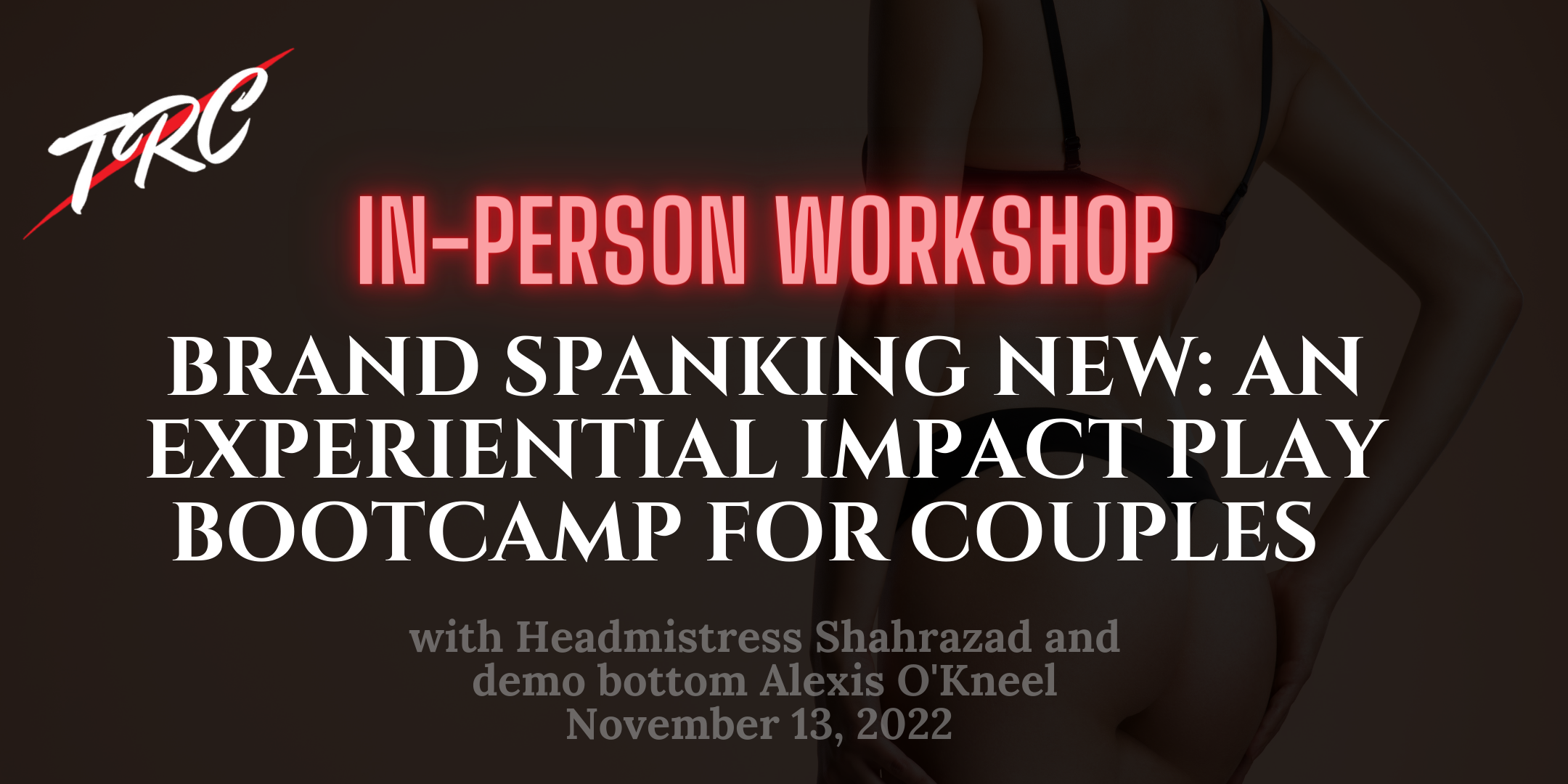The image is an advertisement for an in-person workshop hosted by TRC, titled "Brand Spanking New: An Experiential Impact Play Bootcamp for Couples." The event was held on November 13, 2022. The background is predominantly dark, featuring a grayscale, faint image of a woman seen from behind, wearing black lingerie—a bra and thong underwear. Her left arm rests on her side while her right hand is placed on her hip, accentuating her buttocks. The TRC logo is located in the top left corner, depicted in white with a diagonal red slash. The main text "IN-PERSON WORKSHOP" is prominently displayed in red, with subsequent details in white, stating "BRAND SPANKING NEW: An Experiential Impact Play Bootcamp for Couples." Below this, in gray text, it reads "With Headmistress Shahrazad and Demo Bottom Alexis O'Neill."